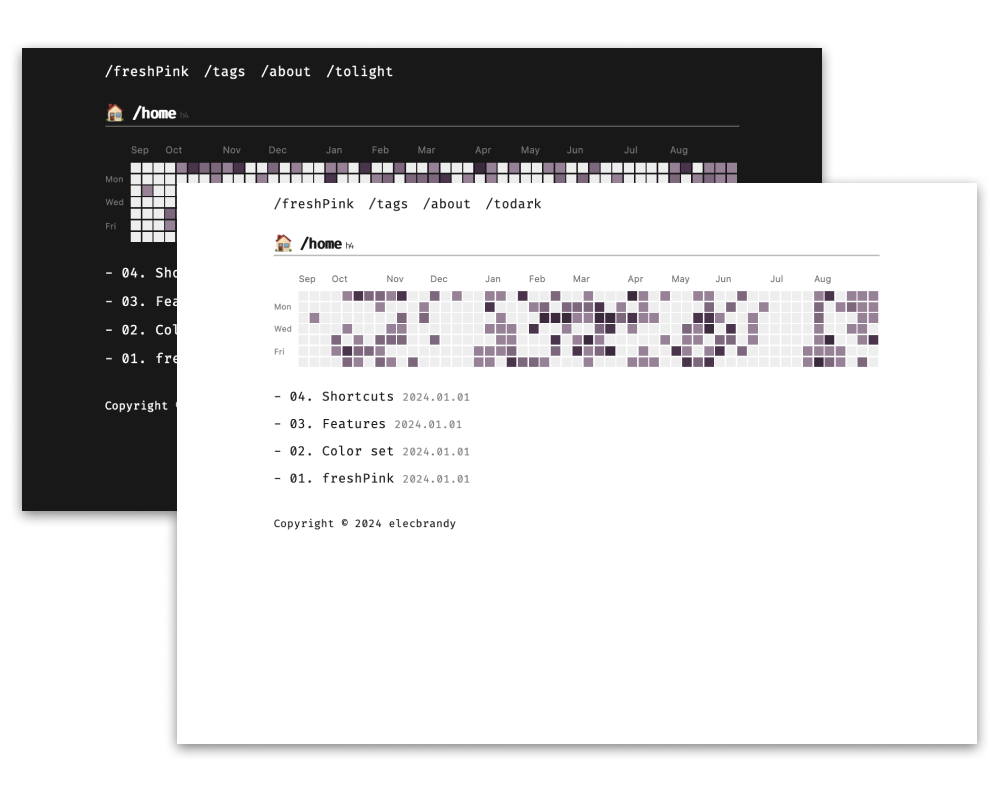The image features a surreal, computer-generated design with a dominant theme of varying shades of pink and purple. At the center, bold white text reads "fresh pink." The background showcases an enigmatic structure composed of multiple shapes and forms, suggesting a chaotic blend of vertical rectangular buildings, spiky elements, and balloon-like structures. This complex amalgamation gives the impression of either an explosion or bubbling crystals, with some parts appearing bulbous and organic. The imagery exudes a pulsating, living quality, further enhanced by the desaturated dark pink backdrop. Overall, the artificial, AI-created design suggests it might be a digital art piece or a placeholder for a modern advertisement. There are no other objects in the scene beyond the central text and the intricate, abstract shapes.